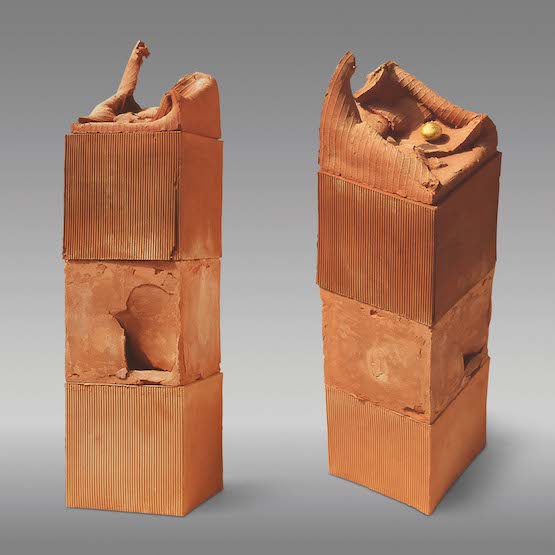This photograph features two almost identical towers made of what appear to be clay cubes, each molded into square shapes with lines running vertically down them. Both structures are composed of three main blocks, with a much-deteriorated fourth block on top. The left tower showcases a middle block that is heavily cracked and dented, revealing the interior. The topmost block of this tower has collapsed into a flattened, disintegrated form. Similarly, the right tower, viewed from a slightly different angle, has a base cube with the characteristic vertical lines, a partially flattened second cube with a minor dent, and a collapsed top block. This top block intriguingly conceals a shiny yellow metal ball, which appears to be an inexplicable addition to the otherwise rugged, earthy constructs. The texture of the material resembles old, dirty fabric, adding to the aged and worn look of the structures. These cubes might evoke images of oversized, heavily weathered packing materials or even the remnants of an ancient game, their state of decay making them both fascinating and slightly grotesque.